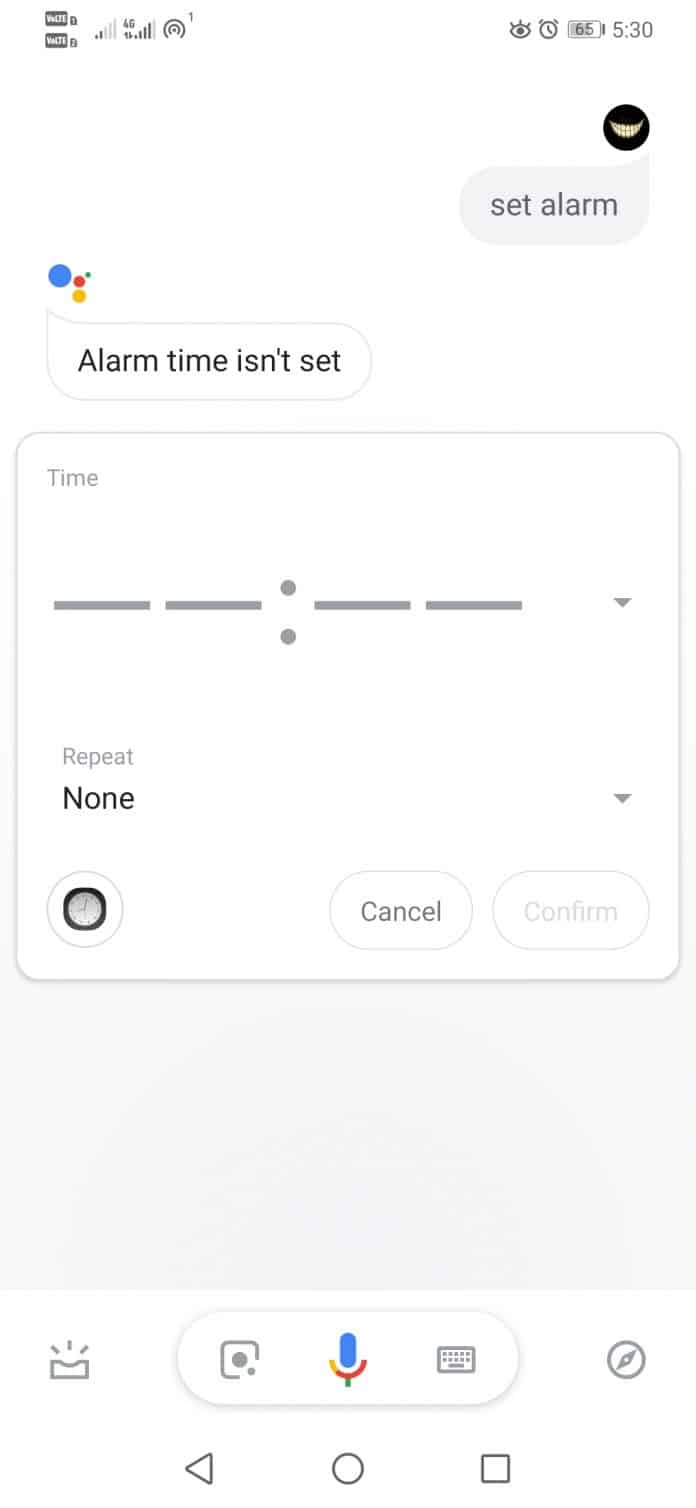This is a screenshot from a Google Pixel smartphone displaying an alarm application. The status bar at the top shows a battery level of 65%, and the current time is 5:30. To the upper right corner, there's a user icon resembling a Cheshire Cat smiling in the dark. 

Beneath the status bar, there is a section labeled "Set Alarm." Below this, you can see a segment that includes Google-related dots: a blue dot, a red dot to its right, a larger yellow dot below, and a small green dot situated 45 degrees above and to the right of the red dot.

The primary section of the screen features a rectangular field with a simple drop shadow. It displays the text "Time: --:--," indicating that no specific alarm time has been set. Below this field, there's a down arrow labeled "Repeat: None," and an inactive "Confirm" button, with a "Cancel" button beside it.

At the bottom of the screen lies the navigation bar, including a microphone icon for Google Voice, a keyboard icon, and what looks like a backward Instagram logo adjacent to stop and play buttons.